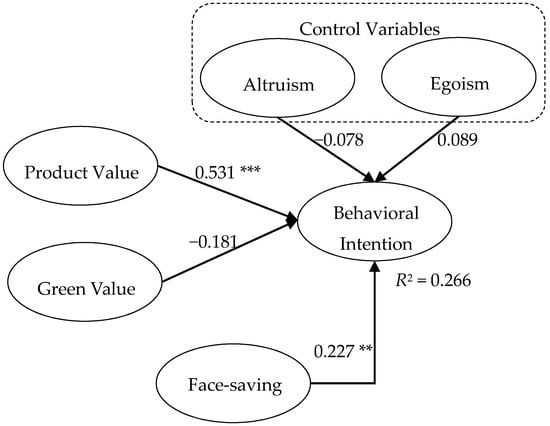The image is a detailed flowchart on a white background, primarily drawn in black ink, outlining various factors influencing behavioral intention. At the top, inside a dashed-line box labeled "Control Variables," are two ovals: one for "Altruism" and another for "Egoism." Altruism has a value of -0.078, and Egoism has a value of 0.089, both connected by arrows pointing to a central oval labeled "Behavioral Intention."

On the left side of the chart are two additional ovals: "Product Value" with a value of 0.531 followed by three asterisks (***), and "Green Value" with a value of -0.181. Both these values are also connected by arrows leading to "Behavioral Intention."

At the bottom of the chart is another oval labeled "Face-Saving," with a value of 0.227 followed by two asterisks (**), also pointing to the central "Behavioral Intention" oval. The overall R-squared value for the model is stated as 0.266, placed just below the "Behavioral Intention" oval. This structured diagram highlights the influence of various factors—altruism, egoism, product value, green value, and face-saving—on behavioral intention, complete with numerical values indicating the strength and direction of these relationships.